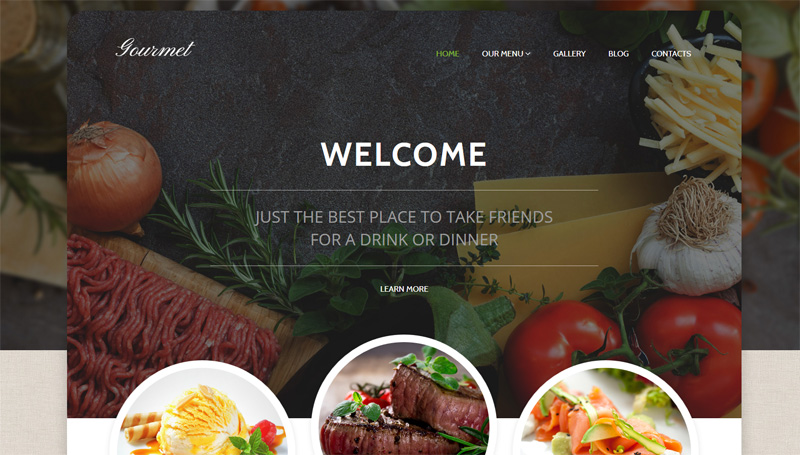A vibrant gourmet food magazine cover showcases a tantalizing array of culinary delights. Central to the image is a steaming bowl of artisanal soup surrounded by an inviting spread. A woven basket displays raw cuts of succulent meat, promising further culinary adventures. The arrangement also features a jumbo onion, luscious ripe tomatoes, and a head of garlic, adding a burst of color and flavor. A side of crisp, golden French fries complements the feast, with sprigs of fragrant rosemary and other spices enhancing the scene. 

The upper left corner proudly displays the word "Gourmet," setting the tone for the sophisticated theme, while navigation options such as "Contacts," "Blog," "Gallery," and "Our Menu" are available for further exploration. A "Learn More" button invites viewers to delve deeper into the offerings of what is described as "the best place to take friends for a drink or dinner."

Inset images within circular frames provide teaser glimpses of additional dishes: a perfectly cooked steak, elegant filet mignon, an artful scoop of fancy ice cream, and a delectable bruschetta topped with cured meats. All of these elements are artfully arranged atop a background image of fresh vegetables, including more tomatoes and aromatic rosemary, adding depth and texture to the composition. 

Overall, this cover is a feast for the eyes, promising an unforgettable gastronomic experience.